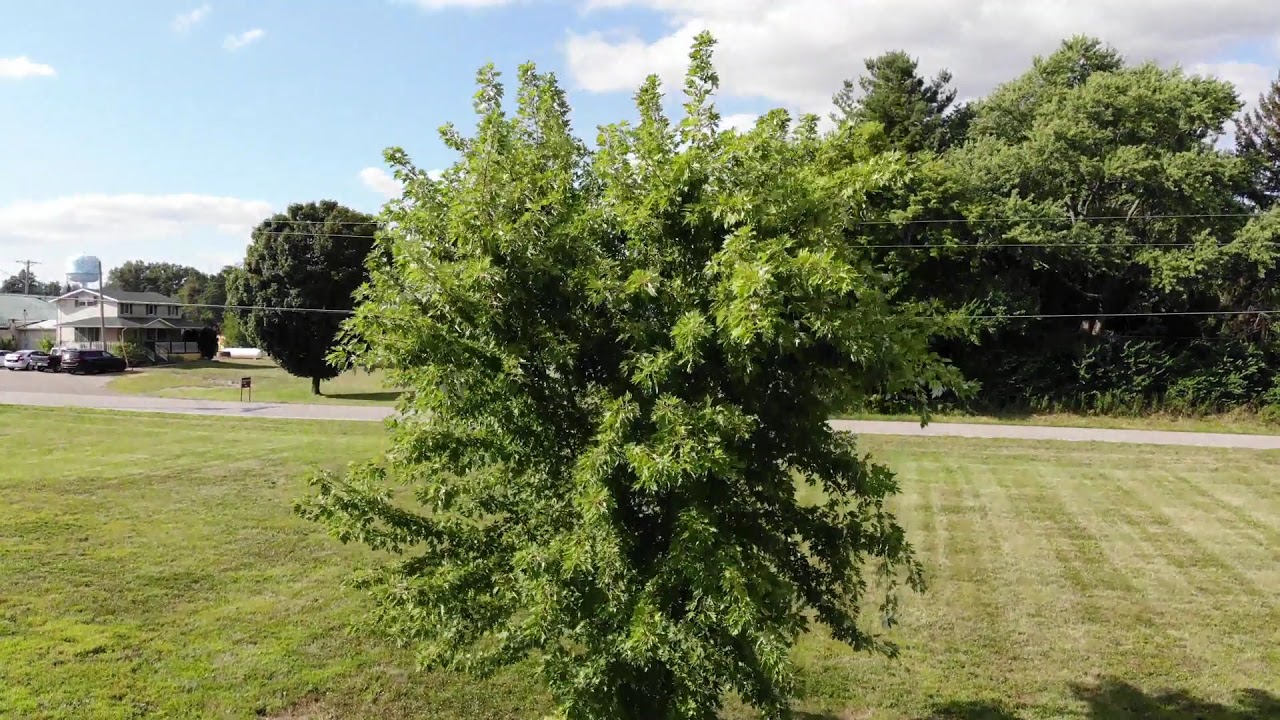A detailed photograph captures a small deciduous tree, densely covered with vibrant green leaves, situated prominently in the foreground of a freshly mowed grassy field. Evidence of the recent mowing is visible in the grid-like patterns left by the lawnmower. The sky above is a light blue, decorated with white and light gray clouds.

In the midground, a paved gray road runs horizontally, cutting through the green landscape from the left to the right of the image. Behind this road is another grass field populated with larger trees exhibiting full green foliage, especially concentrated on the right side. 

To the left of the tree, a white building, possibly a house or small business, stands with a few cars parked in front. The left side of the image also features utility poles and white power lines extending horizontally.

In the distant background, behind the building and trees, a light blue water tower is faintly visible, adding depth to the scene. The entire setting is indicative of a sunny day in a well-maintained residential area, highlighting the neat landscaping and serene environment.